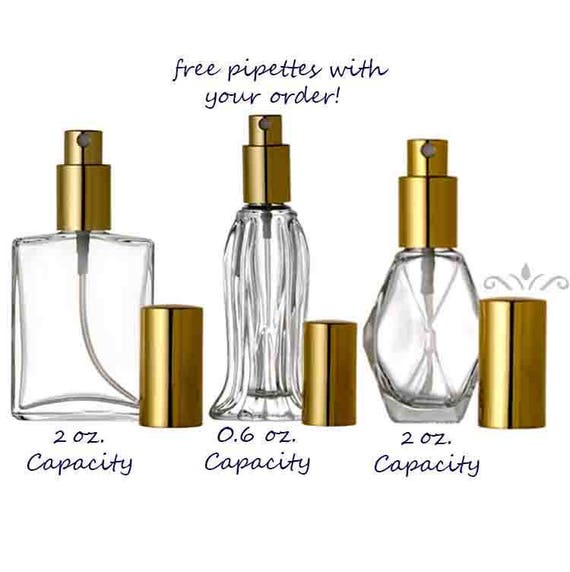This photograph features three distinct clear glass perfume bottles, each topped with a shiny gold spray cap, set against a white background. At the top of the image, a black text reads, "Free Pipettes With Your Order." 

From left to right:

- The first bottle has a two-ounce capacity and is rectangular in shape with a sleek, modern design. It features a gold spray cap and a matching gold lid that covers the sprayer.

- The middle bottle, more decorative and intricate, holds 0.6 ounces. It is slender and tall with a flared base and grooved glass, giving it an hourglass appearance. This bottle also sports a gold spray top and a lid.

- The bottle on the far right has a two-ounce capacity and boasts a unique, multi-faceted shape reminiscent of a marquee diamond with a flat base. It too is adorned with a bright gold spray cap and lid.

These perfume bottles, differing in shapes and capacities, are elegantly arranged to highlight their individual designs and uniform golden accents.